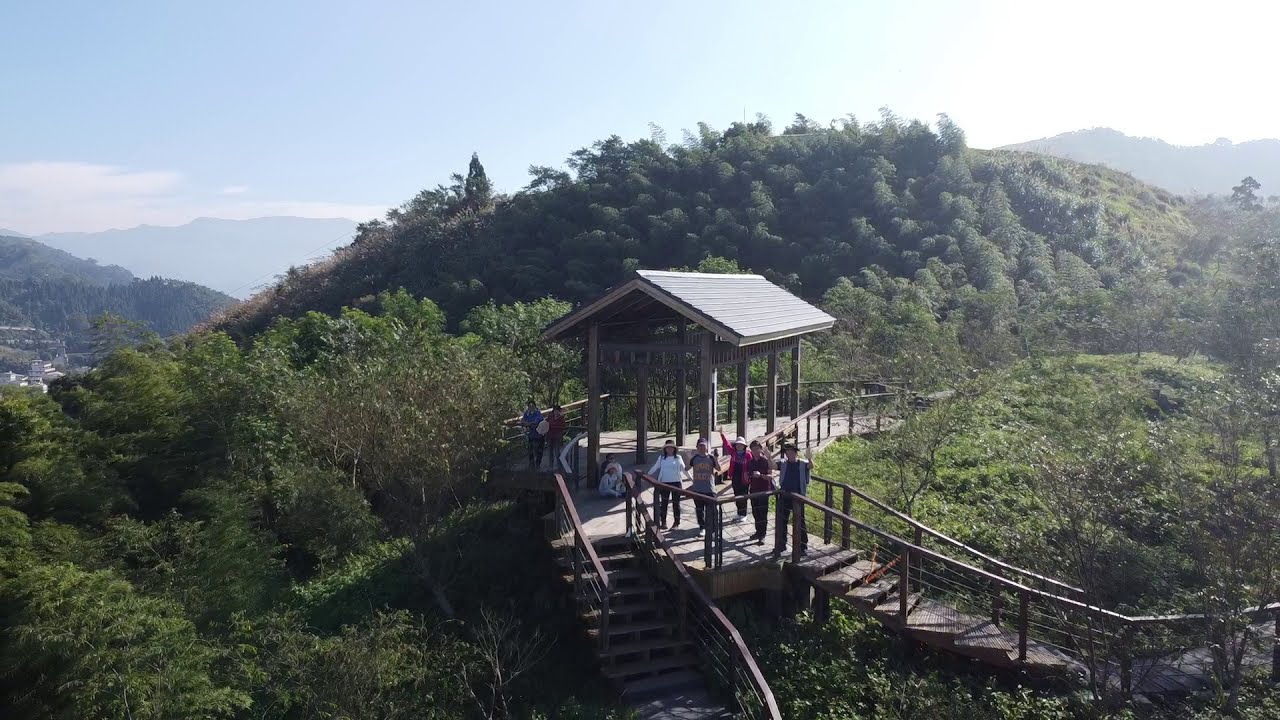The photorealistic image captures an outdoor scene on a bright, sunny day, showcasing a wooden platform above an area teeming with trees and granaries. This platform, composed of brown wood, features multiple staircases leading in and out, and includes a central shaded area with a wooden roof, providing a resting spot for visitors. A crowd of people is gathered closest to the camera, some waving and others posing for a picture. The backdrop reveals a large hill densely covered with vibrant green foliage, swaying gently in the wind, and extending further to reveal more green hills and distant mountainous regions. The scene is framed by additional greenery on both sides, and the clear blue sky, with the sun shining from the right, bathes the entire setting in a warm light, giving a serene yet lively atmosphere. In the far left background, a few buildings suggest proximity to a populated area.